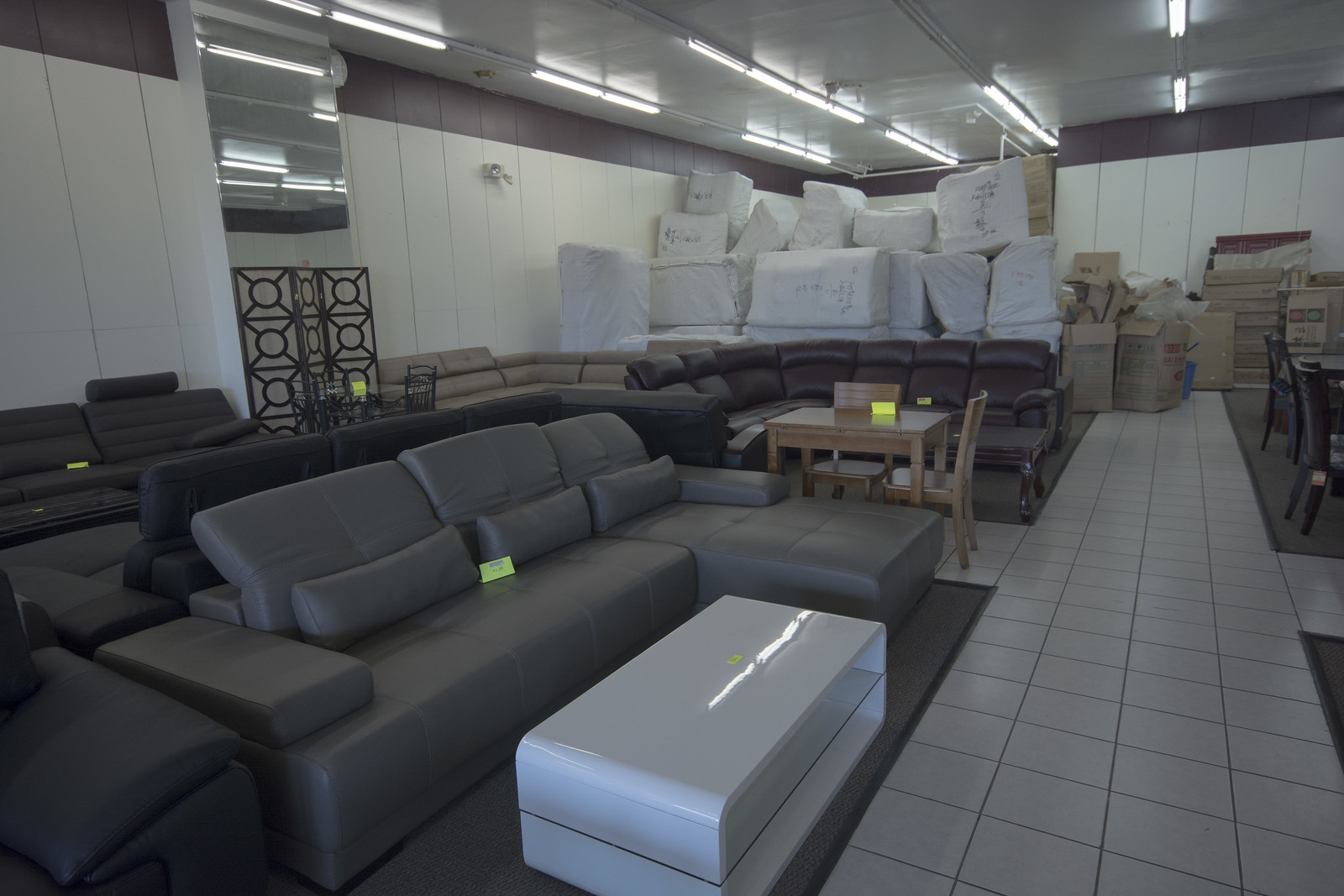This detailed color photograph captures the interior of a furniture showroom or warehouse. The room is lit by long fluorescent tubes installed in the ceiling, which is white just like the broad white panel walls, giving the space a stark and utilitarian feel. The floor is a mix of 10x10 or 12x12 white ceramic tiles forming walkways, and gray carpets in seating areas.

In the foreground of the image is a gray sectional sofa with a small, folded yellow tag, indicating it might be sold. This sectional faces a white ottoman, emphasizing the showroom's modern style. Behind the gray sectional, and back-to-back with it, sits a darker, possibly brown leather sectional that also has padded headrests and appears to be the kind that reclines with the push of a button or pull of a lever.

Along the left side, against the wall, stands a trifold decorative room divider screen. Towards the background, there is a small wooden table flanked by two chairs, and more stacks of cardboard boxes and wrapped furniture pile up to the ceiling, suggesting both showroom and storage functions. White plastic wrap covers many of these items, marked with black marker for identification.

On the right edge of the picture is a glimpse of a dining set, adding more variety to the showroom's inventory. Overall, the photo shows an organized but busy space dedicated to the sale and storage of various furniture pieces, from sectionals to dining sets, all carefully tagged and displayed for potential customers.